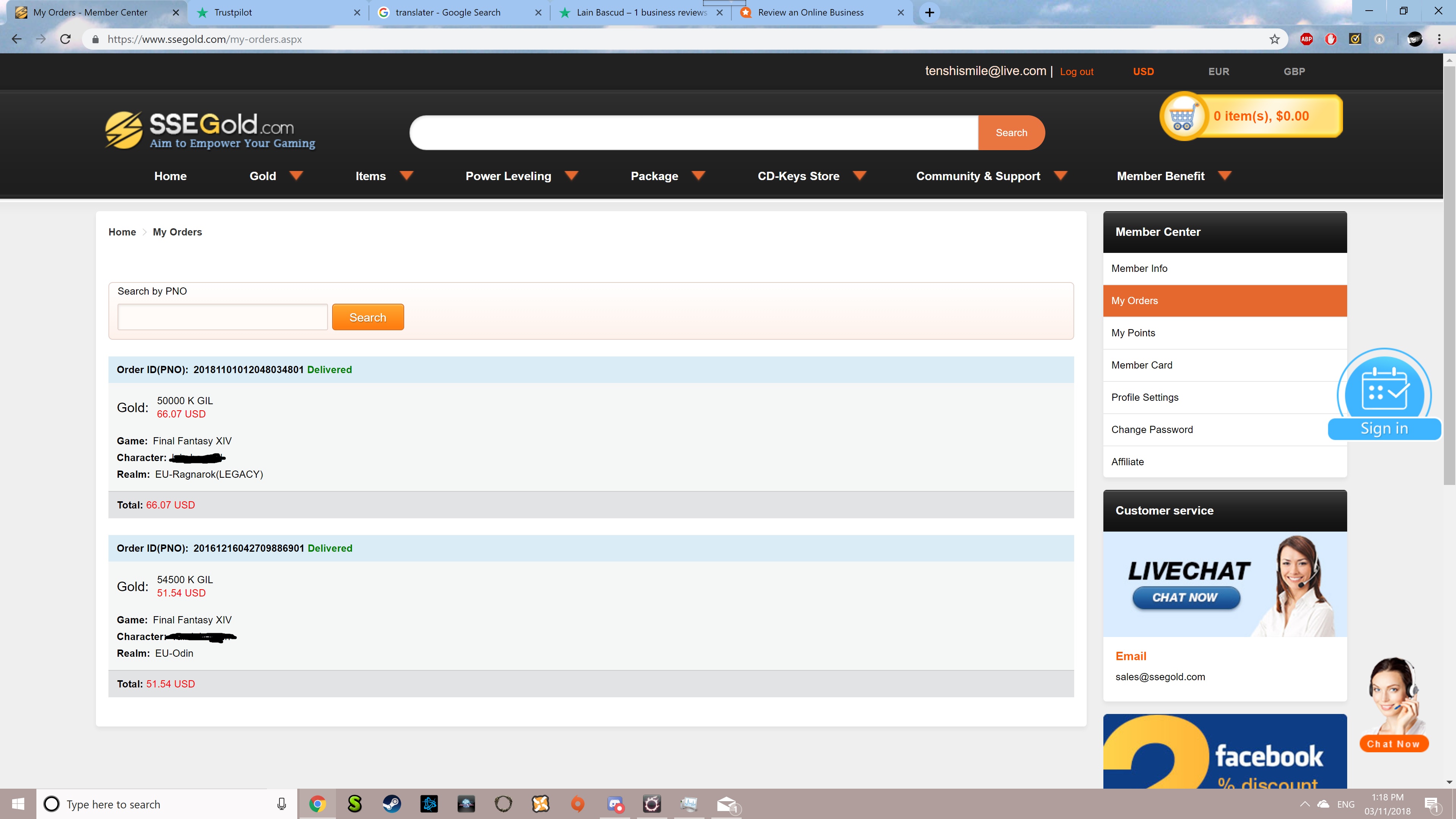This image is a screenshot of the website "ssegold.com," which features the tagline "Empowering Your Gaming." The website specializes in gaming services. Visible on the screen are details suggesting that two orders related to the game "Final Fantasy XV" have been placed, although the specific characters' names are obscured. The prices for these items are displayed in red font, albeit hard to discern due to their small size. Above this window, five tabs are open, but they are unfortunately small and blurry, making their labels difficult to read. On the right side of the screen, a list of options is presented, including live chat, member info, my games, member card, and change password. Additionally, the taskbar at the bottom of the screenshot features several icons, including those for Google Chrome, a messaging application, and an icon resembling a green “S.”